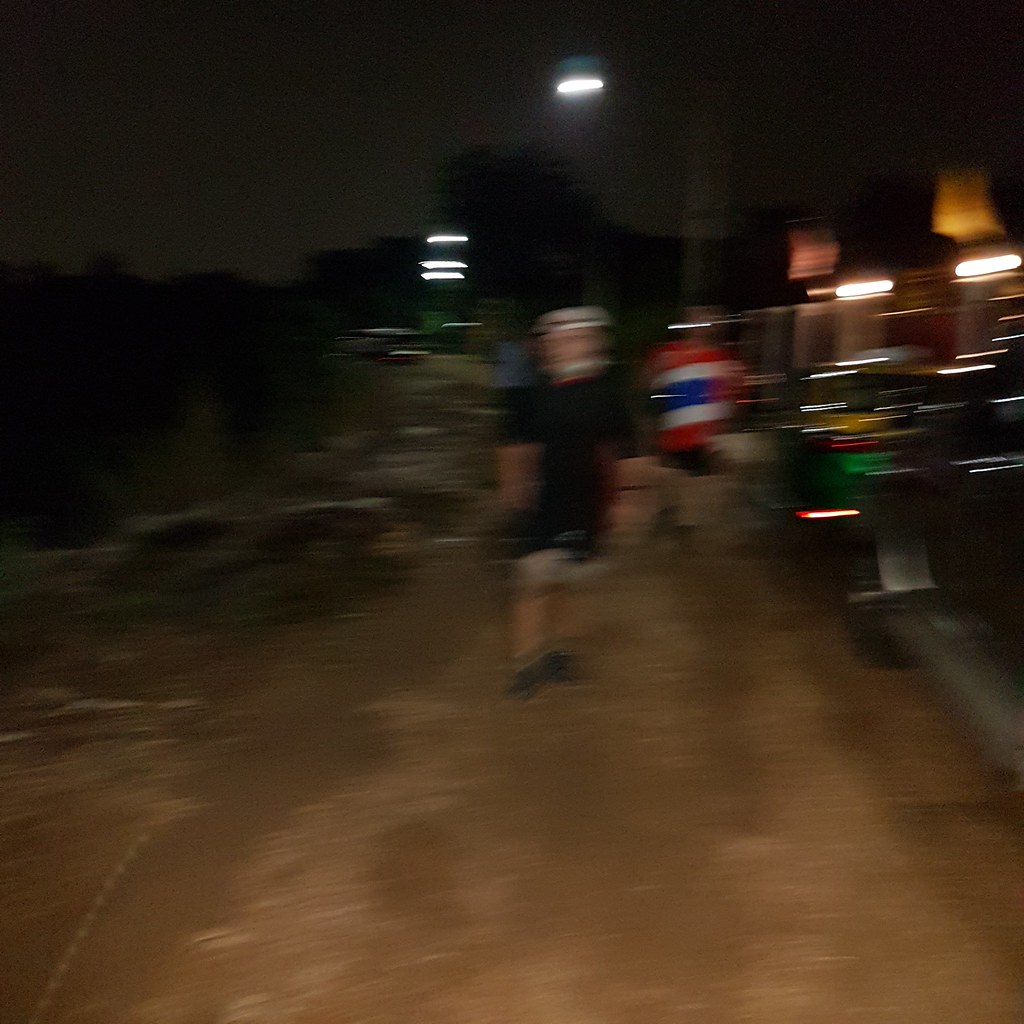In this blurred image, a narrow dirt road or driveway is dimly illuminated by a solitary street light. A man dressed in a black shirt and tan pants walks along the road, sporting a helmet or a silver object on his head. He has just passed another man who is clad in red, white, and blue, appearing to ride a scooter or similar device. To the side, a stone wall partially covered in green vegetation adds texture to the scene. Adjacent to the wall, there is a building that seems to be a restaurant or shop, with a vehicle parked in front of it. The vehicle features green and red elements, and its presence, along with the shop's lights, casts a shiny reflection on the surroundings.